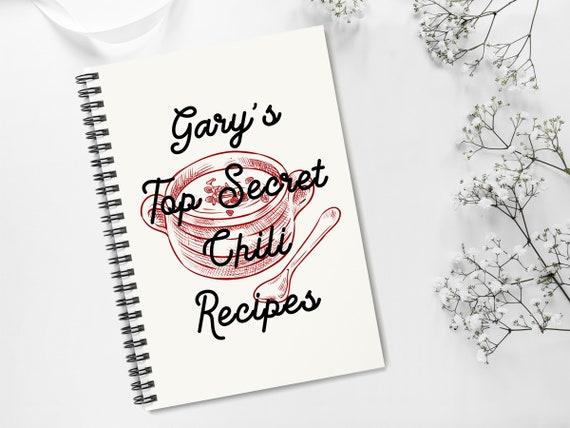The image features a detailed rendering of a book titled "Gary's Top Secret Chili Recipes" on a white counter. The white cover displays the book title in bold, black, cursive font. Below the title, there is a red and white illustration of a chili pot accompanied by a small spoon. The background is a light gray, which contrasts subtly with an oval shadow in a darker shade of gray near the top left corner. Delicate white flowers adorn the right side of the image, extending along the right-hand side and blending into the light gray background. The overall composition suggests a clean and minimalistic design, highlighting the book's title and visuals in a straightforward yet appealing manner.